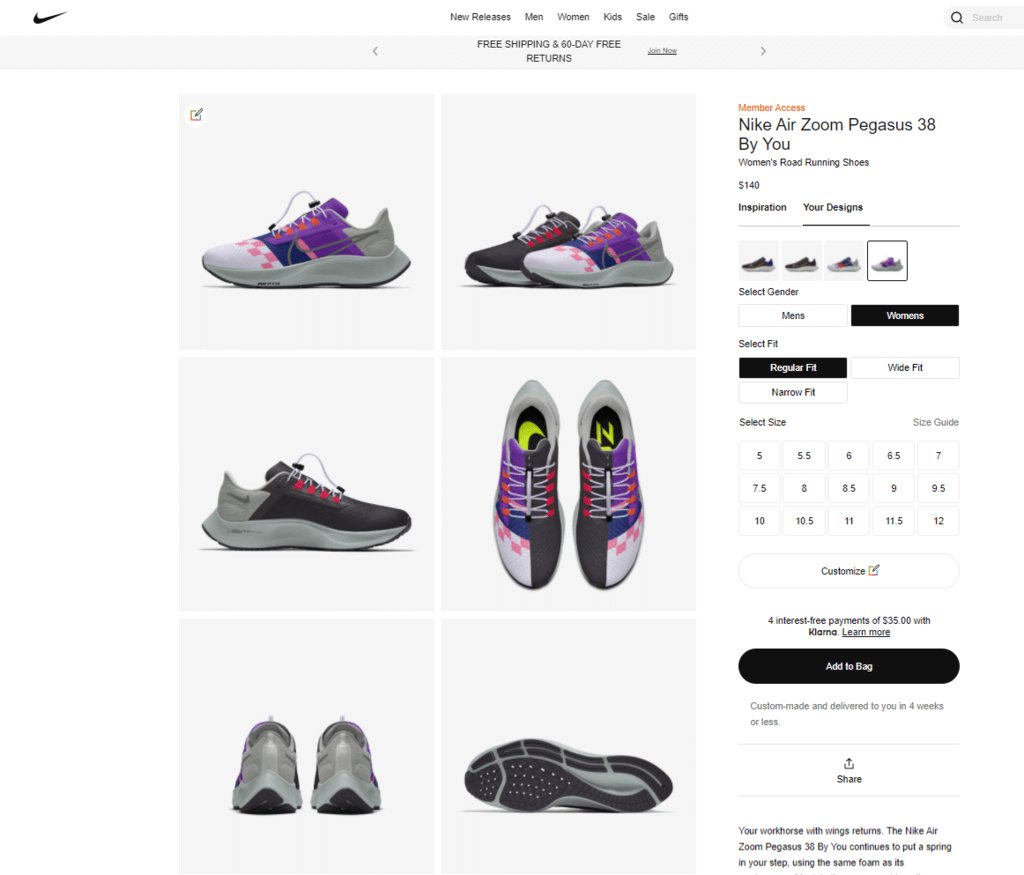Here is a detailed and cleaned-up caption for the image described:

---

This screenshot captures a detailed view of the Nike website, showcasing their "Nike Air Zoom Pegasus 38 by You" women's road running shoes. The Nike logo prominently sits in the top left corner, while a navigation bar at the top lists categories like "New Releases," "Men," "Women," "Kids," "Sale," and "Gifts". Beneath the navigation bar, a banner announces "Free Shipping and 60-Day Free Returns" with a prompt to "Join Now."

On the left side of the page, there is a gallery of six images depicting the shoes from various angles. The first image displays a single shoe from the left side, predominantly white with notable purple accents and red checkboxes. The subsequent image pairs a black shoe beside the previously shown white and purple shoe. The next image features the right side of a black shoe, followed by a top-down view of two white and purple shoes. Below that is a rear view of two shoes in a purplish-gray hue, and the final image shows the sole of a single shoe.

On the right side of the page, text reads "Member Access," introducing the product name and details: "Nike Air Zoom Pegasus 38 by You," priced at $140. Four smaller icons illustrate different color options for the shoes. Options for gender selection highlight "Women's," while options for fit show "Regular Fit" as highlighted, alongside choices for "Wide Fit" and "Narrow Fit." Size options range from 5 to 12, including half sizes.

At the bottom, buttons display options to "Customize" and "Add to Bag." There's also a note indicating payment flexibility with "Four interest-free payments of $35 with Klarna."

---